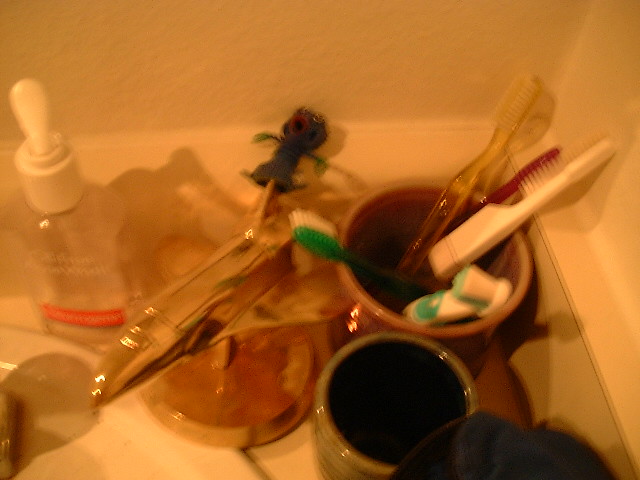This is a poorly lit, blurry photograph, likely taken with a cell phone, depicting the cluttered corner of a bathroom countertop near a sink. The entire image has an orange or peach-colored hue due to overhead lighting. In the foreground, a ceramic cup with a black interior holds an assortment of five toothbrushes in various colors and designs: see-through, red, white, turquoise and white, and green. Next to the cup, a lid or possibly another container lies on the countertop. A black, cartoonish figure appears on top of a hand or face wash bottle. The white edge of the sink is barely visible in the bottom left corner. Additionally, a dark green towel and a greenish cup can be seen in the bottom right corner. The top right-hand corner shows the countertop meeting the wall, which has a pinkish-white tint. The overall composition is chaotic and hard to discern due to the blurriness and poor lighting.